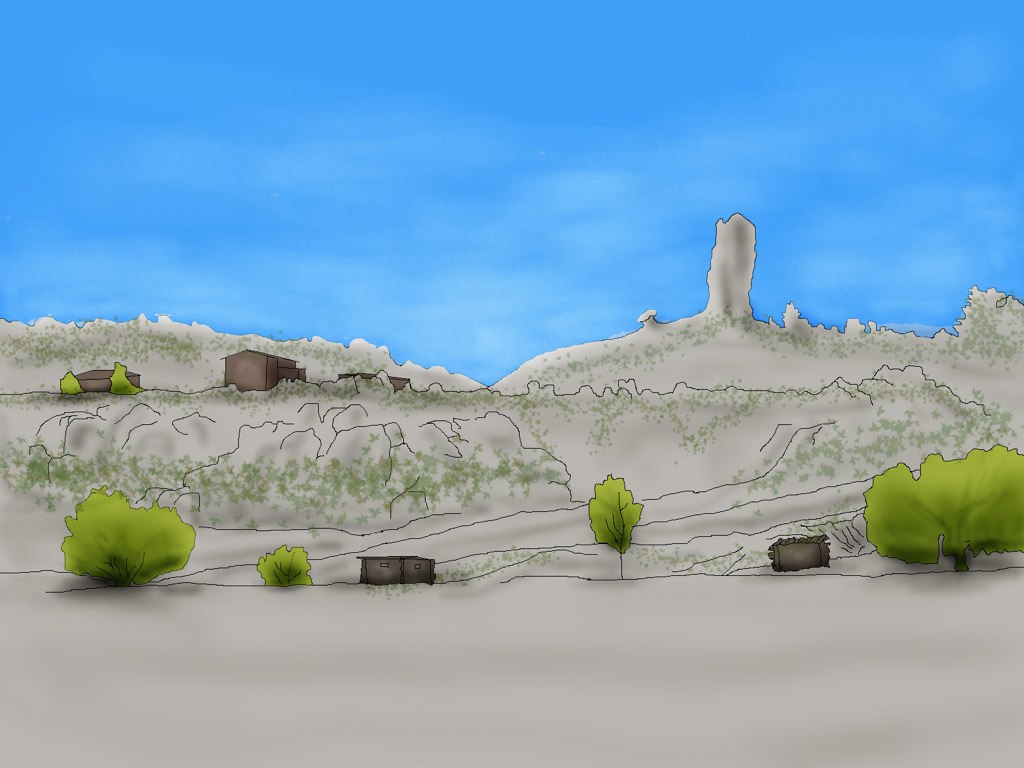This detailed watercolor painting depicts a cartoonish desert landscape under a vivid blue sky mottled with wispy white clouds. The foreground is flat, covered in sand, and features a mixture of green vegetation, including two small bushes, a taller shrub, and a tree to the right. Additionally, there's a wooden wagon turned over, hinting at a rustic, perhaps abandoned setting.

In the mid-ground, a ridge emerges with a few small gray buildings, possibly outbuildings or shelters of some sort. To either side of these buildings, there are clusters of green shrubbery. The terrain then transitions into a rocky, rough hillside adorned with patches of grasses and shrub-like plants. Atop this hillside, towards the left, sits a cluster of larger structures resembling homes, suggesting the outskirts of a desert town. Beside one of these buildings are additional green shrubs.

Further back, a prominent monolithic rock formation rises, accompanied by several smaller rock pillars, creating a dramatic focal point against the skyline. Overall, the painting balances natural arid elements with human-made structures, capturing the essence of a sparsely vegetated, rugged desert scene.